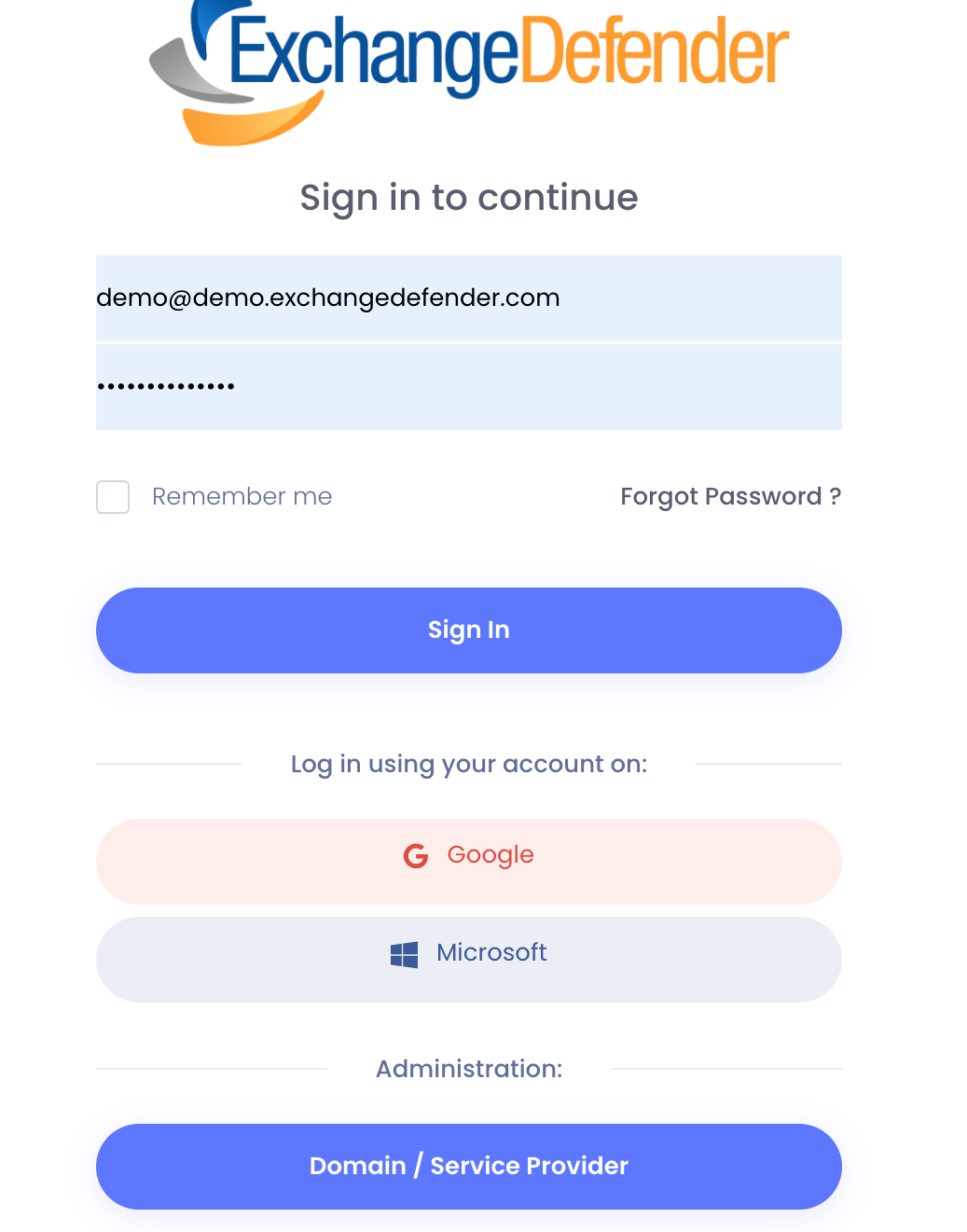A detailed screenshot of a login page is depicted, apparently taken from a user's computer or phone screen. The top heading prominently features the words "Exchange" in blue and "Defender" in orange. Just beneath this heading, the screen prompts the user with "Sign in to continue." 

Directly below, there are fields for entering a username and password, each outlined with a light blue border. Adjacent to the password box, a small square checkbox labeled "Remember me" is available for users who wish to save their login details. To the right of this checkbox is a link labeled "Forgot password?" in a similar light blue font.

Further down, there is a solid light blue oval button with the caption "Sign in" written in white letters at its center. Below this sign-in button, an additional instruction reads in gray text: "Log in using your account on." Accompanying this text are two large buttons for alternative login options. The first is a light pink rectangle with the word "Google" in a bold orange font, while the second is a light gray rectangle with "Microsoft" indicated.

At the bottom of the page, the word "Administration" is displayed, followed by another light blue oval button bearing the white-lettered text: "Domain/Service Provider." The layout and design elements suggest a professional and user-friendly interface designed to accommodate various login preferences.